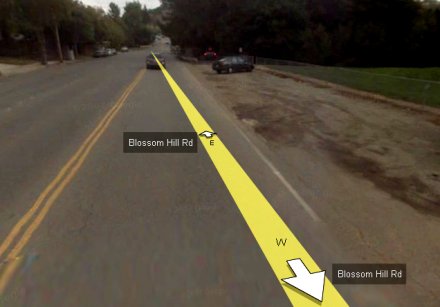A detailed screenshot captured from a GPS or map service on a PC, showcasing Blossom Hill Road. The name of the road is clearly indicated in the center and at the bottom of the screen. A prominent yellow line bisects the street, guided by two directional arrows pointing east and west, signifying the road's two-way traffic. Additionally, the street itself features two yellow lines, denoting a caution or no-passing zone. On the right side of the road, a car is parked unconventionally against the flow of traffic on the swale area. Another vehicle is seen traveling eastward in the foreground. The surroundings are lush, with trees adorning both sides of Blossom Hill Road and well-maintained grass enhancing the right side of the view.